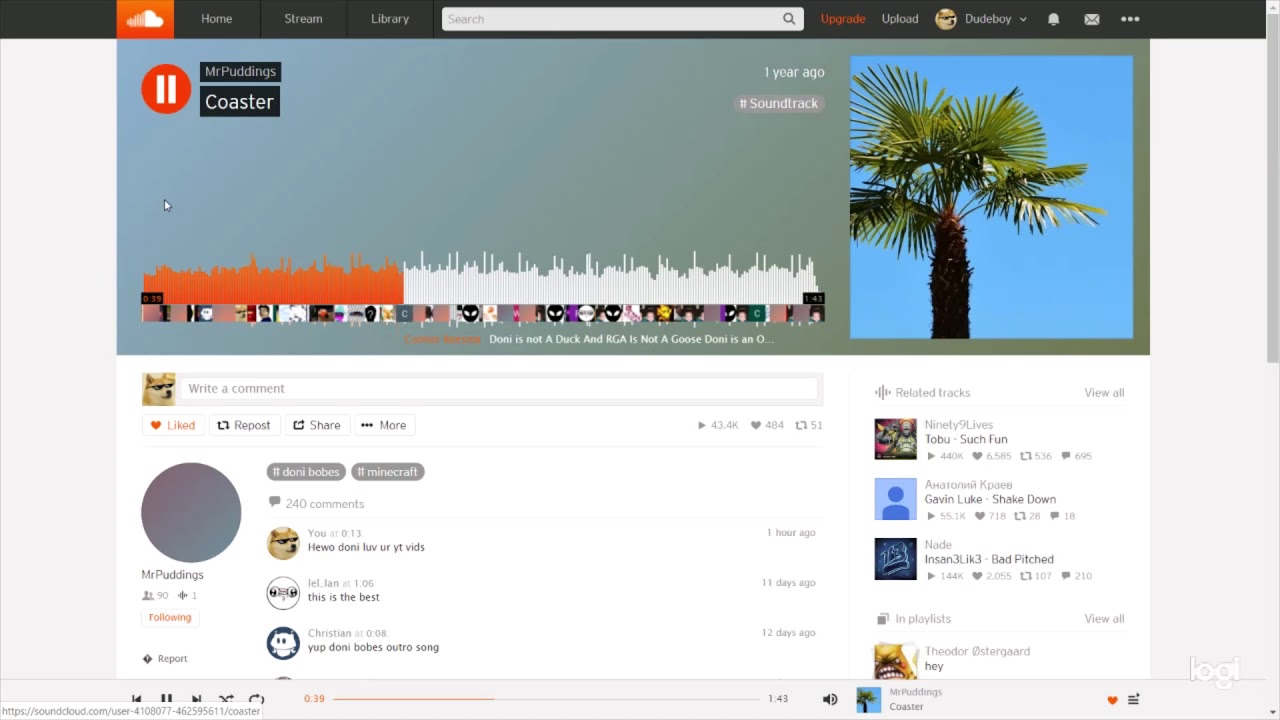The image showcases a detailed interface of a digital music and social media platform. At the top, a black header contains navigation elements, including a home button, stream, and library options, alongside a search bar. A red notification labeled "update" and buttons for uploading and a dash function are visible. On the right side of this header, there are icons: a small circle with a dog's picture, a bell, an envelope, and three dots (likely for additional options).

Below this header, the page has a light gray backdrop and features a large gray content box. Within this box, an orange circle with two white lines is displayed prominently beside two black circles labeled "Mr. Postings" and "Coaster." To the right, text indicating "one year ago" and "soundtrack" is visible. 

Further down, the interface displays a visual representation of sound waves in orange and white lines and an assortment of small images under it. A blue box showcases an image of a palm tree against a light blue sky, emphasizing a serene aesthetic. 

A large white box is present on the page featuring another small dog's picture and an empty white box labeled "write a comment" with a gray background. Additional interactive elements include options such as a red heart labeled "liked," repost, share, and more actions. 

Beside this, a big gray circle with some text beneath it, several gray buttons, and elements related to "Minecraft" in red are seen. There are three comments timestamped as "one day ago" and "two and a half days ago." 

On the right-hand side, under "related tracks," there is an option to "view all" and four images along with names and brief information about the tracks. At the bottom of the page, a gray box encompasses various icons, a red progress line with a number on one end, and a gray number on the opposite end. The section at the end also features another small image of a palm tree, a red heart, and three gray lines, indicating additional options or interactions.